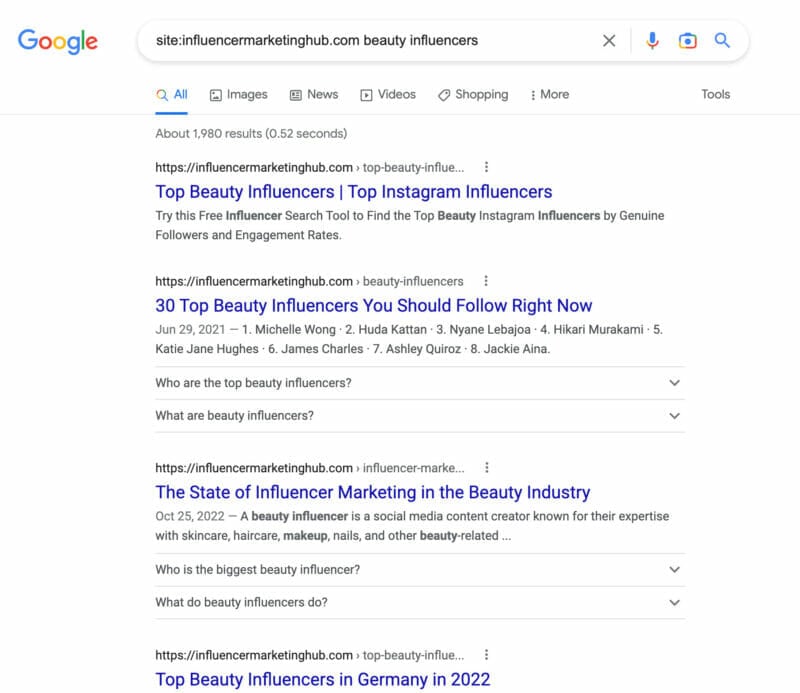A user performed a search on a computer using Google, illustrated by the Google logo on the left of the search bar. They searched for "site:influencermarketinghub.com beauty influencers" which resulted in various relevant articles and lists. The first result was titled "Top Beauty Influencers, Top Instagram Influencer" and included a free influencer search tool to find the top beauty Instagram influencers based on genuine followers and engagement rates. The second result, "30 Top Beauty Influencers You Should Follow Right Now," listed the top eight influencers with their names highlighted. Following this, there was an article about the state of influencer marketing in the beauty industry, explaining that a beauty influencer is a social media content creator specializing in skincare, hair care, makeup, nails, and other beauty-related topics. Further down, another result posed questions such as “Who is the Biggest Beauty Influencer?” and “What Do Beauty Influencers Do?”. The final noted result was titled "Top Beauty Influencers in Germany in 2022." This summarized the search results displayed on the computer.